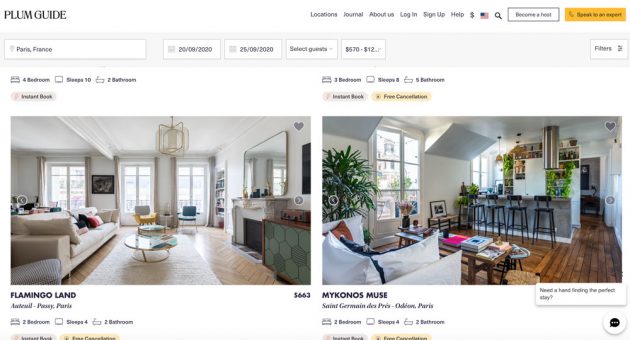A detailed view of a real estate guide on a minimalist white webpage with elegant black text, showcasing interior photographs of two apartments. In the top left corner, the website name "Plum Guide" is prominently displayed, while the top right features user-friendly search fields for locations, property addresses, price ranges, and availability periods.

The center of the guide presents vibrant color photographs of the interiors of two distinct apartments. The left image highlights an apartment with a sophisticated palette of gray, neutral, and white tones, exuding a serene and modern vibe. In contrast, the right image showcases another apartment adorned with chic white furnishings and complemented by sleek black bar stools positioned in front of a stylish gray kitchen counter. The warm wooden flooring adds a touch of rustic charm to this space. Both living areas in the photographs appear immaculate and minimalistic, creating inviting and stylish environments. The second photograph further features an open kitchen concept, seamlessly integrating the living space and kitchen, reflecting modern design principles.